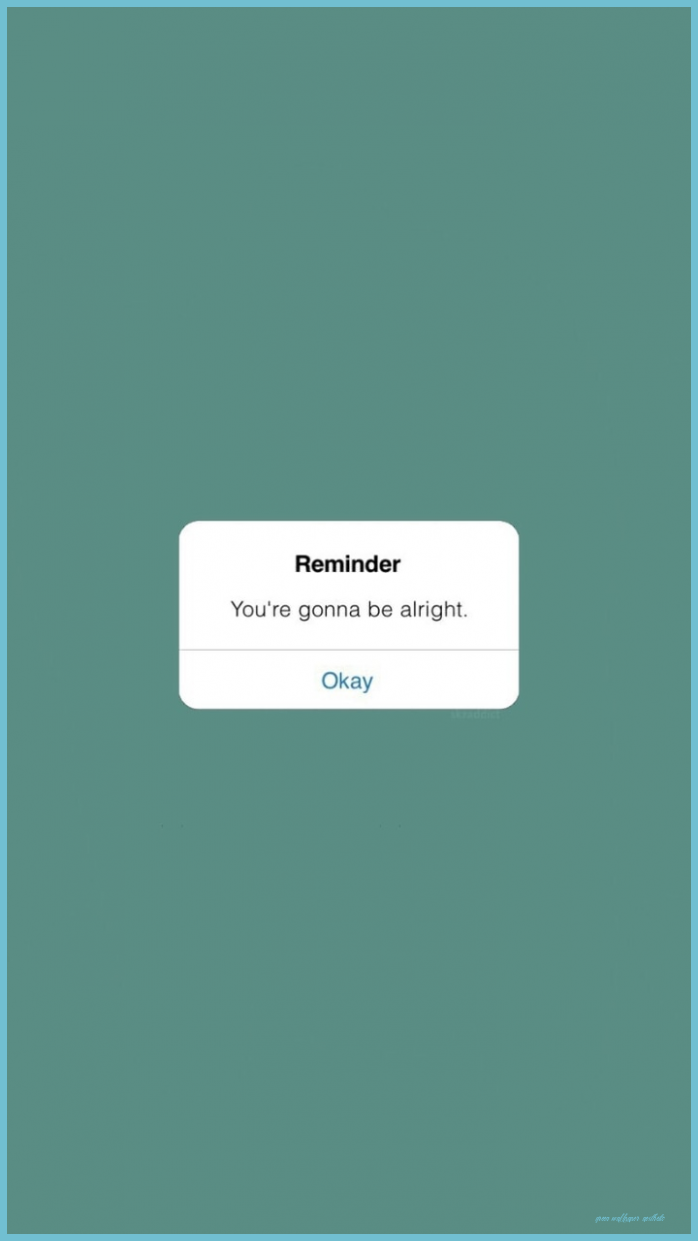A teal rectangle with a light blue border encases the image. At the center, a white rectangle is positioned horizontally with its shorter sides at the top and bottom. The word "REMINDER" is prominently displayed in bold letters at the top of the white rectangle. Beneath this, the text "You're going to be alright" is inscribed in a lighter font. A light grey line separates this reassurance from the word "OK," which is written in blue letters that match the border color. The initial "O" is uppercase, while the remaining letters are lowercase. The image is simple and uncluttered, featuring shades of blue and white with minimal black and blue text. It's the kind of uplifting message commonly found on positivity-focused blogs or as a personal note of encouragement between friends.